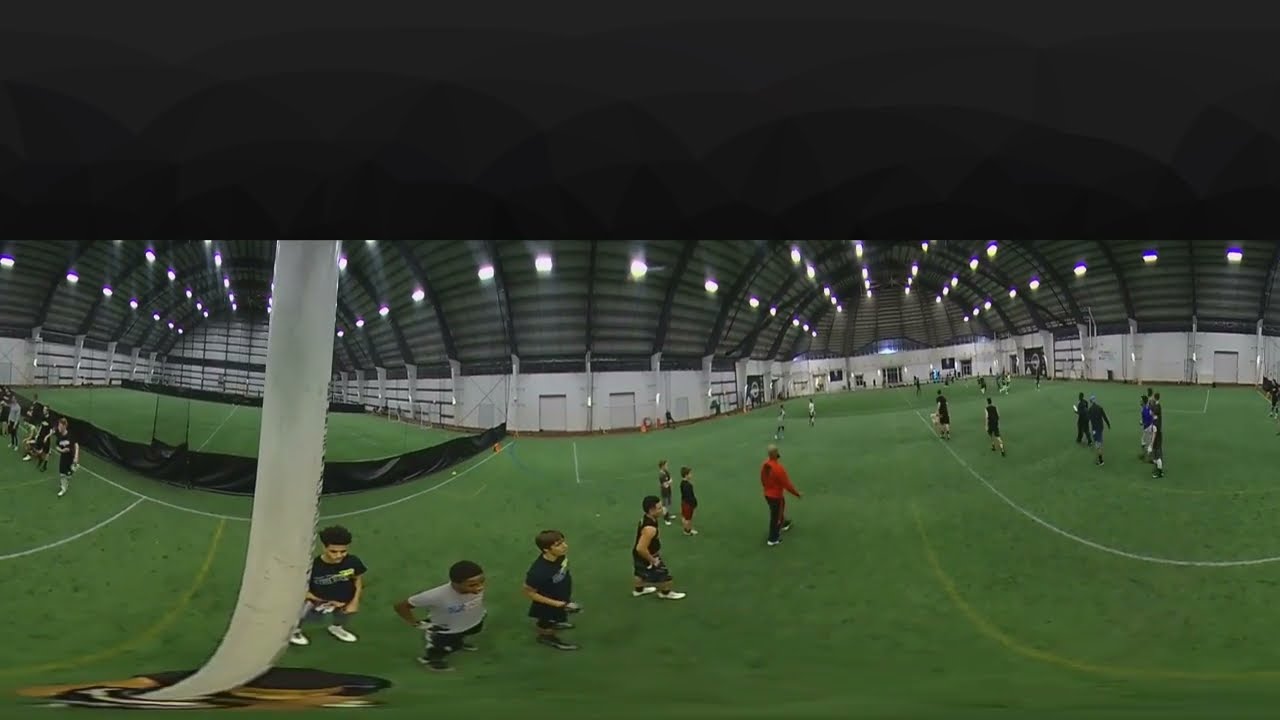The image is a panoramic shot of an indoor recreational center with a domed, arched gray ceiling supported by black metal beams. The camera captures a 360-degree view that makes the entire scene curve unnaturally, allowing the viewer to see from the front entrance to the back of the facility. The walls are white, and the ground is covered with bright green turf marked by white and colored lines demarcating different sections of the playing field.

Bright and shiny white lights line the sides of the building, illuminating the area. On the right side of the image, a large indoor playing field is occupied by numerous people, primarily young athletes, all wearing athletic shirts, shorts, and sneakers, suggesting they are engaged in sports practice, possibly soccer. In contrast, the field on the left side of the image, partitioned by black fabric fences, is empty. A prominent black barrier further sections off part of the field on the left side. The scene is bustling with activity, yet somewhat disorganized, as some individuals seem to be running while others walk across the turf. A figure in a red shirt, possibly a referee, is also visible among the athletes. Overall, the image captures the dynamic and vibrant atmosphere of an indoor sports facility.